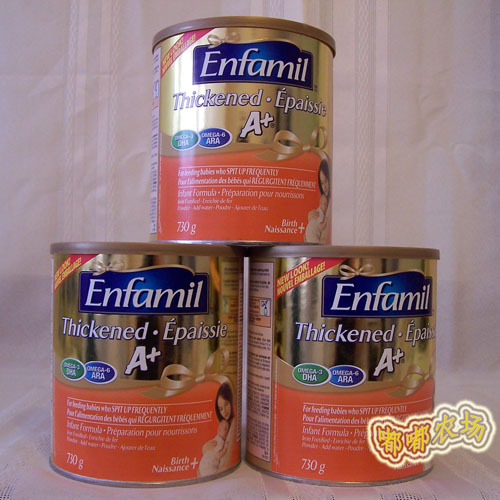The image features a fabric background with vertical white lines. In the foreground, there are several items of clothing. Prominently displayed is a stack of infant formula containers. The container at the top has a gold lid and transitions into an orange base. The top-left area of the container features a red label with yellow text and an adjacent window containing blue text on a white background. On the left side of the container, there is a thick, opaque green circle, and on the right side, a blue circle. Both circles contain white text that is difficult to fully discern but possibly mentions the frequency of use and the word "infer formula." The bottom left corner of the label indicates "730 grams," while the bottom right corner states "birth, nascence," next to an icon depicting a woman hugging a baby. The label suggests the formula is specifically designed for babies who spit up frequently and includes information in multiple languages, potentially including French.